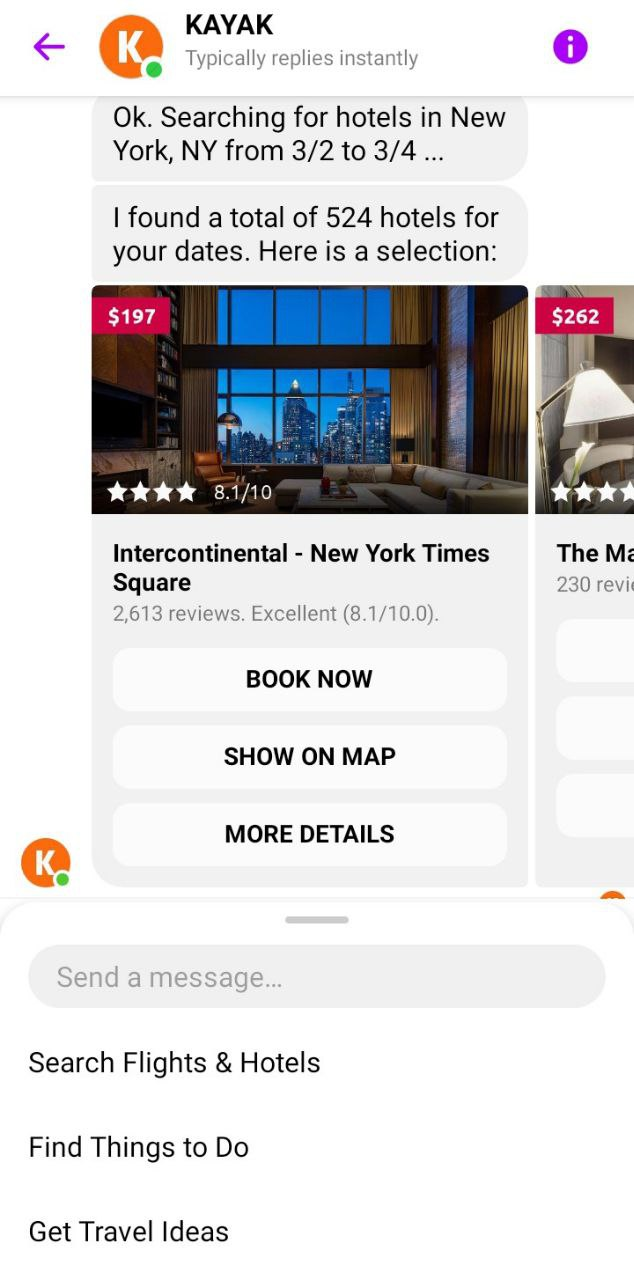**Detailed Screenshot Description**

On the left-hand side of the smartphone or tablet screenshot, there is a purple arrow pointing to an orange circle that contains a bold white letter "K." Adjacent to the orange circle is a small green circle. Following these icons, bold black text reads "KAYAK." Directly underneath "KAYAK," in gray text, it states "Typically replies instantly."

On the right-hand side of the screenshot, there is a purple circle with a white "I" inside it. Below this icon is a section showcasing a correspondence, part of which is displayed in gray and black text that reads: "Okay, searching for hotels in New York, NY. From 3/2 to 3/4…" This is followed by another comment, "I found a total of 524 hotels for your dates. Here is the selection…"

Next, a hotel listing is displayed, featuring a large lobby with a brown chair on the left-hand side, gray couches, and large windows offering a cityscape view. The hotel has a 4-star rating, shown in white stars, and an 8.1 out of 10 rating displayed in white text. In the top left-hand corner of this hotel listing, there is a red rectangle with a dollar sign and the number "197," indicating a rate of $197 per night. Below this price, bold black text reads "Intercontinental – New York Times Square." Directly underneath, gray text notes "2,613 reviews," followed by the word "Excellent" and an 8.1 out of 10 rating in parentheses.

Below the hotel description are three light gray oval buttons with bold black text. The first button says "Book Now," the second says "Show on Map," and the third says "More Details."

On the right-hand side of the screenshot is another hotel listing that includes a white lampshade. A red rectangle displays "$262," followed by "230 REB," which is cut off. At the top of this listing, bold black text reads "The MA."

In a new section of the screenshot, the orange circle with a white "K" and a green circle appears again, indicating the person is online. A chat bubble is visible, shaped as a dark gray oval, with darker gray text inside that reads "Send a message." Underneath, bold black text says "Search flights and hotels. Find things to do. Get travel ideas."